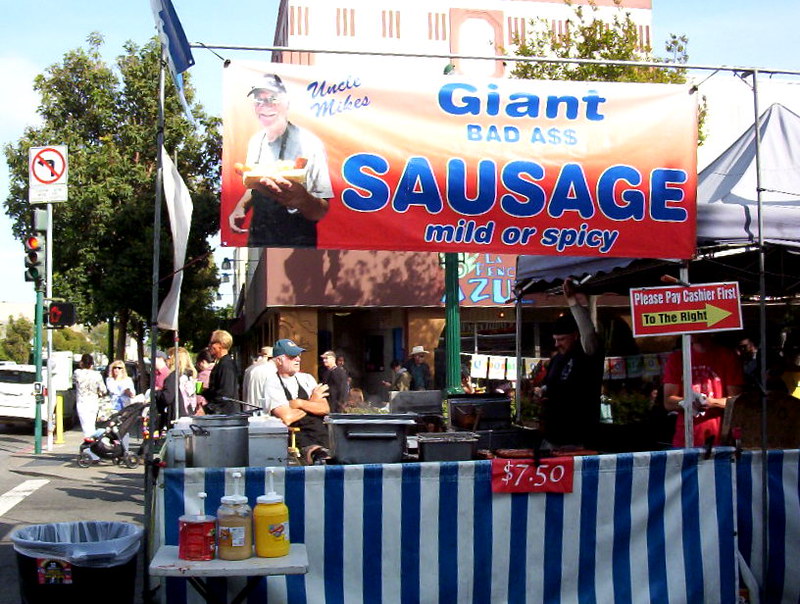This image captures a bustling outdoor food stand set up at the corner of a busy intersection with a stoplight, featuring Uncle Mike's concession area prominently. The stand is adorned with a vibrant red banner at the top, displaying an older man, presumably Uncle Mike, holding a hot dog and smiling. Next to his image in bold blue text, the banner reads "Uncle Mike's Giant Badass Sausage: Mild or Spicy," with the word "ass" humorously replaced by two dollar signs. Below this main banner, blue and white vertical striped canvases surround the stand, adding to its distinctive look.

To the left of the stand, there's a small table with condiments like ketchup, mustard, and possibly relish, along with a trash can. A smaller sign underneath the banner instructs, "Please pay cashier first," with a yellow arrow pointing to the right. Another prominent feature is a red sign with white lettering that announces the price of the sausages as $7.50.

The background reveals a street, a large building, trees, and people walking by, indicating that this concession stand is set up in a lively, busy area. The stand appears to be open-air with no actual roof, showcasing kitchen equipment visible behind Uncle Mike.